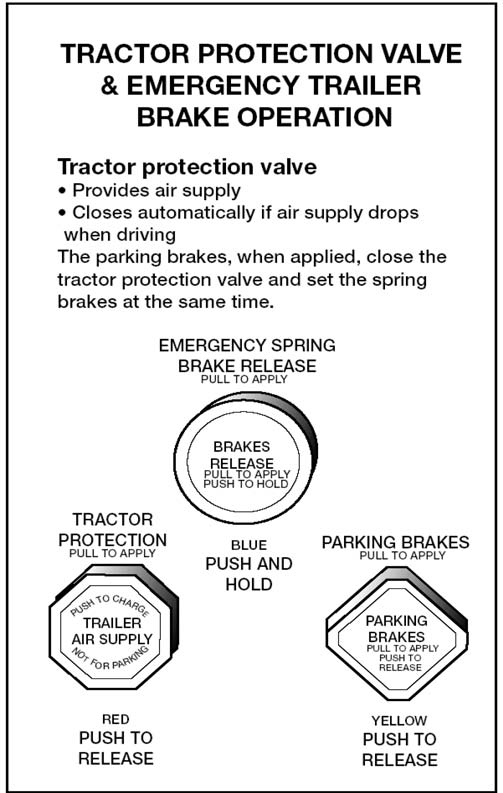The image is an informational brochure with a white background and black text explaining the Tractor Protection Valve and Emergency Trailer Brake Operation. The title at the top reads "Tractor Protection Valve and Emergency Trailer Brake Operation." Below this, it states that the Tractor Protection Valve provides air supply and automatically closes if the air supply drops while driving. Another text describes how the parking brakes, when applied, close the tractor protection valve and simultaneously set the spring brakes.

Beneath this textual information are three detailed figures. 

1. The top figure features a circular button with the label "Emergency Spring Brake Release, Pull to Apply." Inside the circle, it says, "Brakes Release, Pull to Apply, Push to Hold."

2. The bottom left figure is an octagonal button labeled "Tractor Protection, Pull to Apply." Inside the octagon, it reads, "Push to Charge Trailer Air Supply, Not for Parking." Below this octagonal figure, the text reads, "Red, Push to Release."

3. The bottom right figure is a diamond-shaped button with a caption above it saying, "Parking Brakes, Pull to Apply." Within the diamond, it states, "Parking Brakes, Pull to Apply, Push to Release." Below this figure, it reads, "Yellow, Push to Release."

The entire brochure is bordered by a thin black line, adding a clean frame to the detailed instructions and illustrations provided.